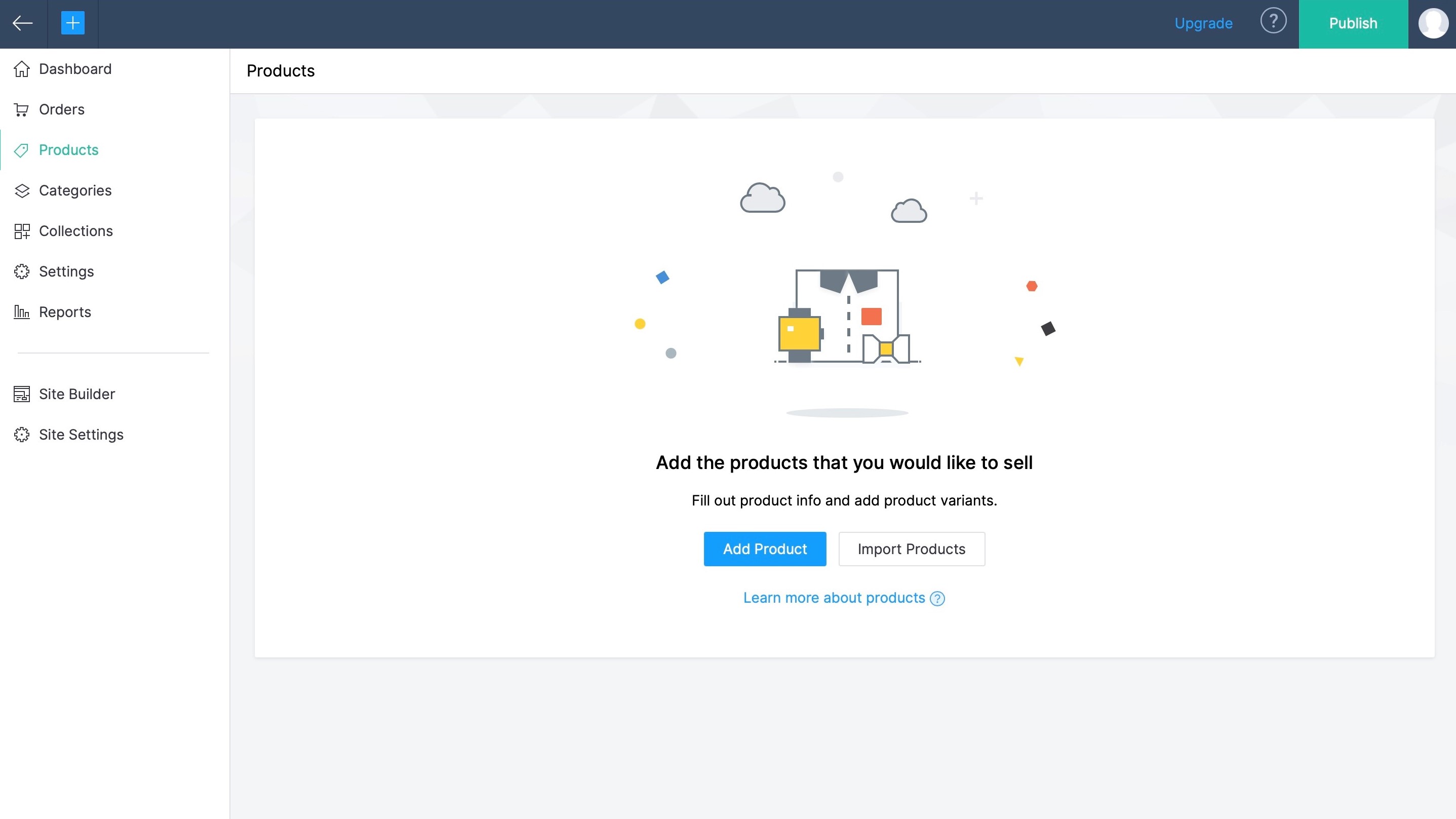Description of the E-Commerce Website Interface:

At the top of this e-commerce website, a long, dark blue rectangular bar spans the width of the page. On the left-hand side of this bar, there is an arrow pointing to the left, followed immediately by a plus sign enclosed within a light blue box. Moving to the right along the bar, the word "Upgrade" is prominently displayed, followed by a small question mark icon encased in a circle. Next, there is a prominent green button labeled "Publish," and finally, a user icon is positioned on the far right.

The main body of the website features a clean, white background with subtle gray highlights. Positioned in the upper left corner, the word "Dashboard" is clearly visible. Beneath the "Dashboard" title, a vertical menu lists several options: Orders, Products, Categories, Collections, Settings, and Reports. Further down, separated by a light-colored horizontal bar, additional options for "Site Builder" and "Site Settings" are present. 

In this particular view, the "Products" tab is highlighted, indicating that this is the active page. The central content area is titled "Products," and just below this title, there is instructional text that reads: "Add the products that you would like to sell, fill out product info, and add product variants." Below this guidance text, there are two prominent buttons: a blue "Add Products" button and a white "Import Products" button.

Towards the bottom of the page, a small logo is visible. This logo features various items such as a bow tie, a shirt, a smartwatch, and some clouds, providing a visual representation of different product categories available on the site.